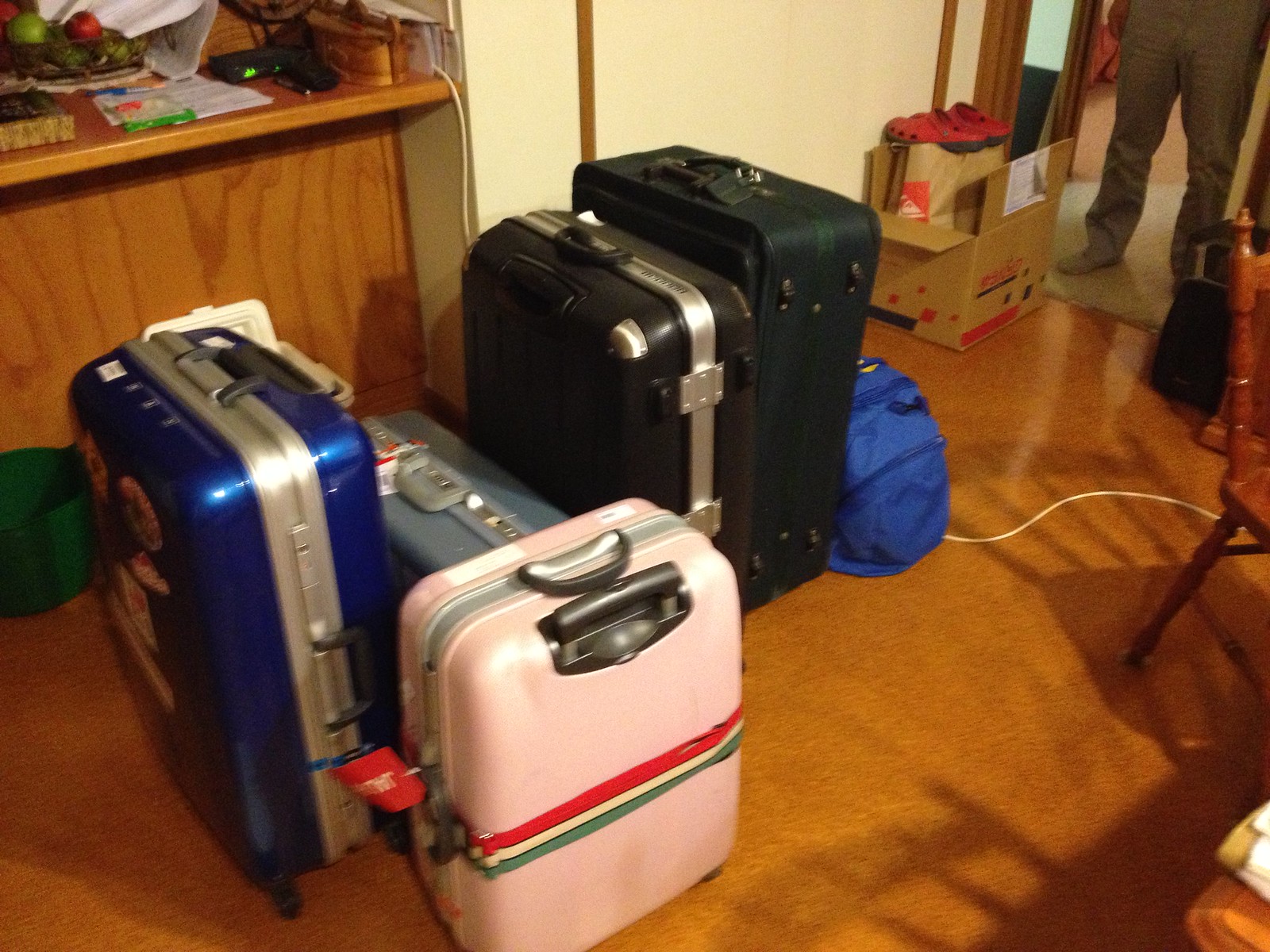In this detailed indoor scene, the image showcases six pieces of luggage arranged on a medium-hued wooden floor. Prominently positioned are a blue duffel bag and five assorted suitcases: a royal blue hard-sided one with a front design, a small light blue-gray piece, and a distinctive white hard-sided luggage adorned with three horizontal stripes in green, medium beige, and red, complete with a red tag. Also visible are a black hard-sided suitcase trimmed with silver and a hunter green soft-sided luggage. Beside the luggage sits a cardboard box topped with a pair of red shoes. In the background stands a man, with only his gray socks and pants visible. The floor, possibly hard vinyl, contrasts with the cluttered yet orderly arrangement of personal belongings, hinting perhaps at a move or a trip. Additional details include a hint of furniture and items such as a chair, a shelf with fruit, a router, and various miscellaneous objects against white walls trimmed with brown lining in the background.